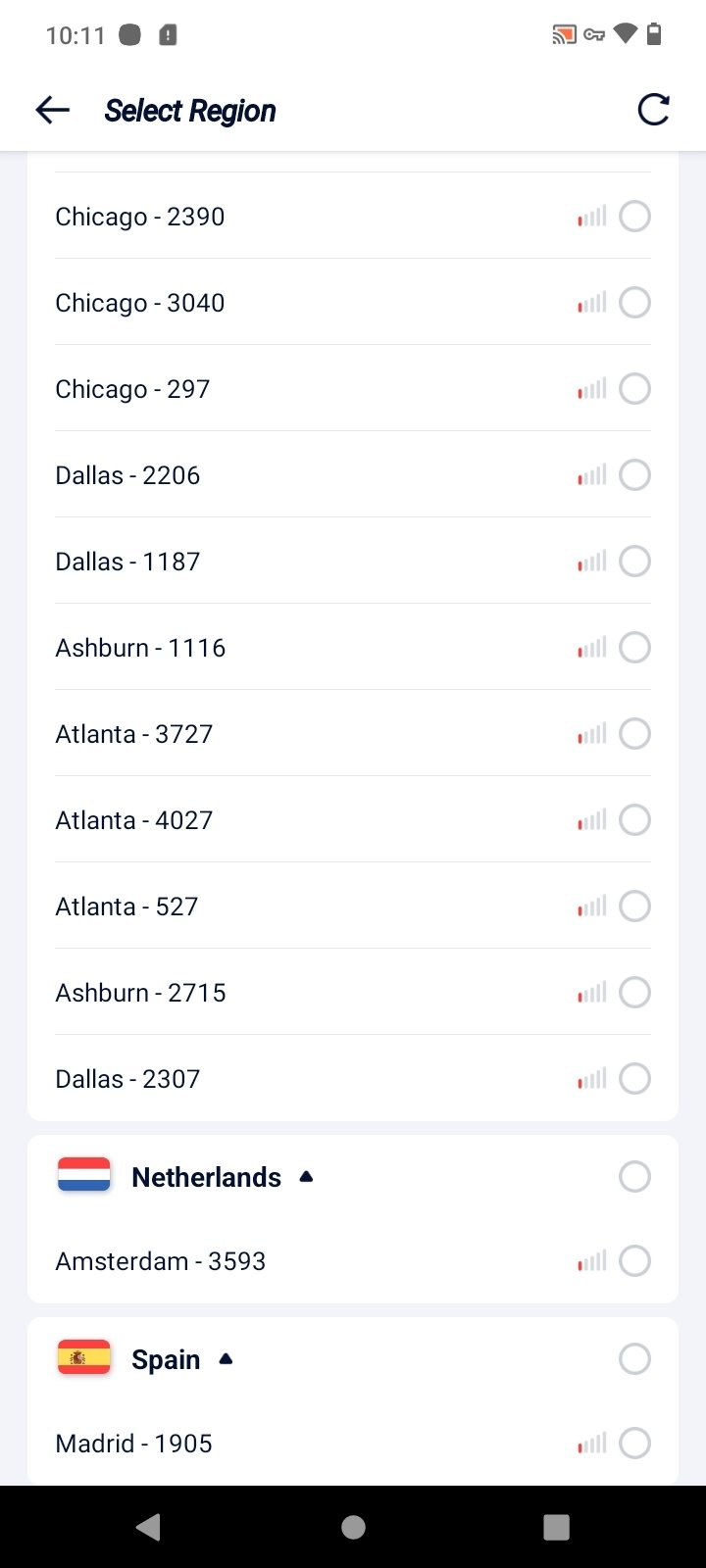This image is a screenshot from a cell phone. In the top-left corner, the time reads "10:11," and the top-right corner displays Wi-Fi and battery icons. Below this, the header "Select Region" is present. The next section lists various cities with corresponding region codes and radio buttons to the far right of each entry, none of which are selected. The cities and codes include:

- Chicago 2390
- Chicago 3040
- Chicago 297
- Dallas 2206
- Dallas 1187
- Ashburn 1116
- Atlanta 3727
- Atlanta 4027
- Atlanta 527
- Ashburn 2715
- Dallas 2307
- Netherlands (flag icon) Amsterdam 3593
- Spain (flag icon) Madrid 1905

The image is purely textual and does not contain any photographs, people, animals, birds, plants, flowers, trees, buildings, bridges, or automobiles. The orientation of the screenshot is taller than it is wide.